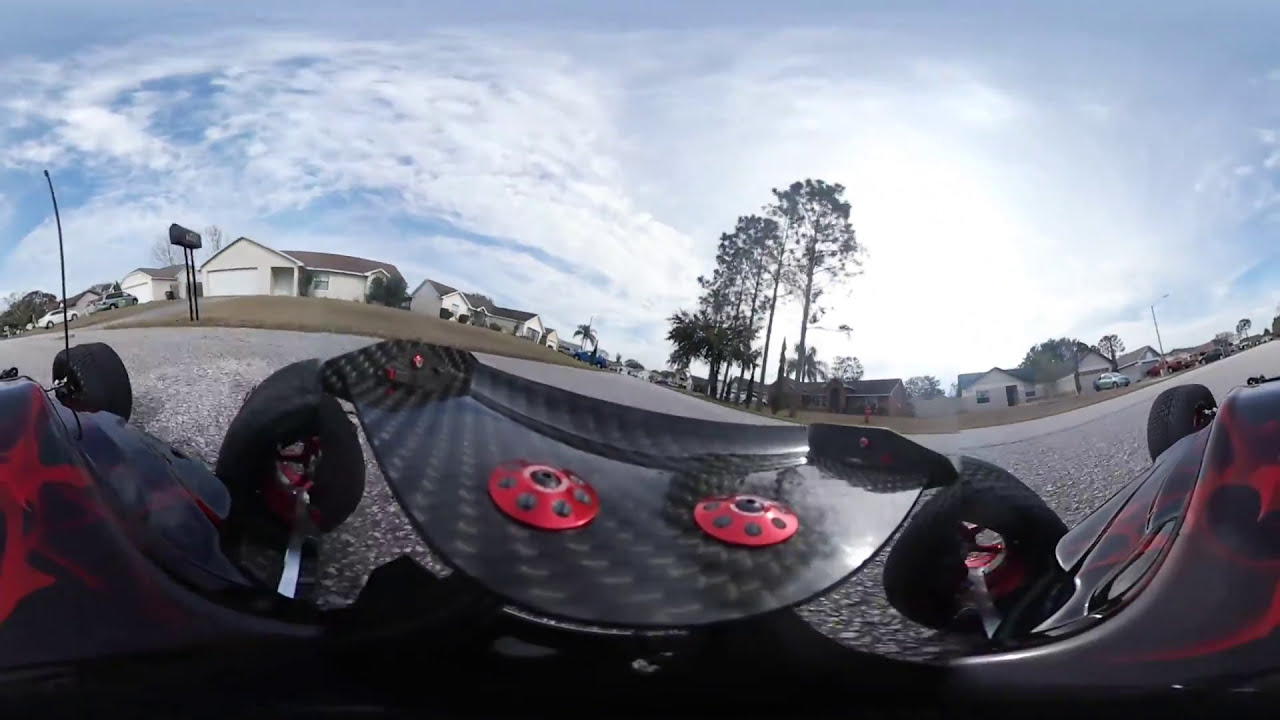The image features a panoramic, 360-degree view showing a warped and wavy scene. At the foreground, there's a red and black vehicle that looks like a cross between a car and a go-kart, possibly a motorcycle or four-wheeler. The vehicle has a carbon fiber front with red flames painted on it and visible tires sticking out on both sides. The surrounding environment is a bland suburban neighborhood with light tan, single-story houses with brown roofs lining a blacktop road. There are garages with driveways in front of these houses. On the right-hand side of the street, several large trees, including palm trees, are in view, full of leaves at the top. The sky above is broad with scattered clouds, presenting a washed-out blue hue, perhaps during sunset. There are some yards with dried-up, brown grass, a few vehicles, and mailboxes in front of the homes, giving the scene a somewhat deserted appearance. Two small, red details, possibly parts of the vehicle, add a slight contrast to the otherwise monotonous landscape.